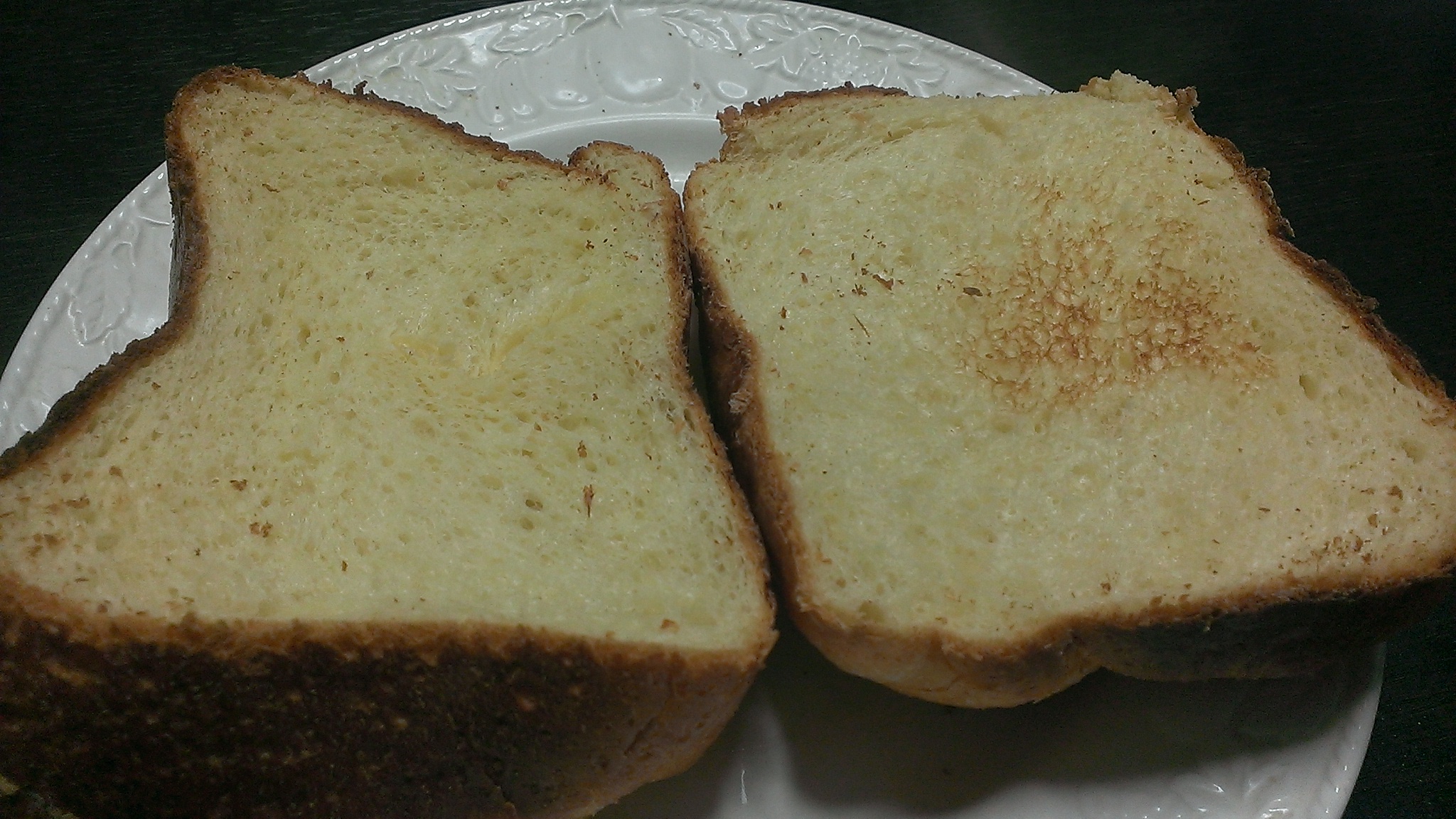The image features a close-up photograph centered on two slices of thick toasted white bread, both resting on a smaller white plate. The bread displays hints of golden to dark brown coloration, indicative of toasting, with patches of yellow suggestive of butter having been applied. The slice on the right shows slightly darker spots, implying it was closer to burning. The plate itself has a glossy finish and features a subtle floral and leaf embossing around its border. The background is predominantly black, perhaps a black tablecloth, which starkly contrasts with the plate and bread, drawing focus to the toast. The image is captured from a perspective that gives an intimate view of both the top and side edges of the bread, emphasizing its thickness and texture.